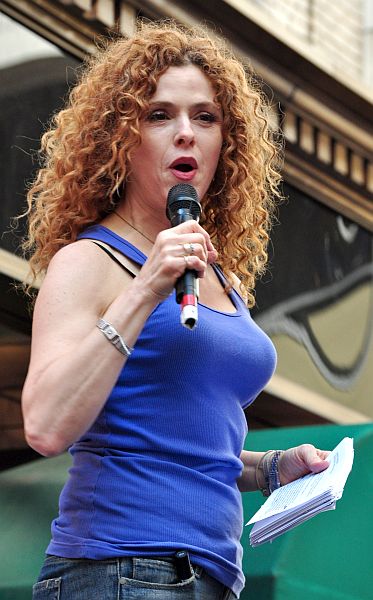This is a photograph of a Caucasian woman with curly red shoulder-length hair, styled casually and parted in the middle. She is wearing a blue ribbed tank top with a tan bra strap visible on the left. Her right arm, which appears slightly muscular, holds a black microphone with a red and white stripe near its base, and she wears a silver bracelet on the same arm. On her right hand, a silver-colored ring adorns her long, unpolished fingernails. The woman's lips are painted with red lipstick, and her eyes may feature eyeshadow. She holds a stack of small, white papers in her left hand, while wearing blue jeans, which are visible at the bottom of the image. Behind her is a green canopy structure, suggesting an outdoor setting, possibly on a stage in front of a building. The background includes various diagonal elements: a row of what resembles white spools beneath white, sunlight-illuminated Venetian blinds, followed by black bands, and a carved wooden border. The overall background composition appears complex and layered with dark and teal green sections, adding to the depth of the photograph.